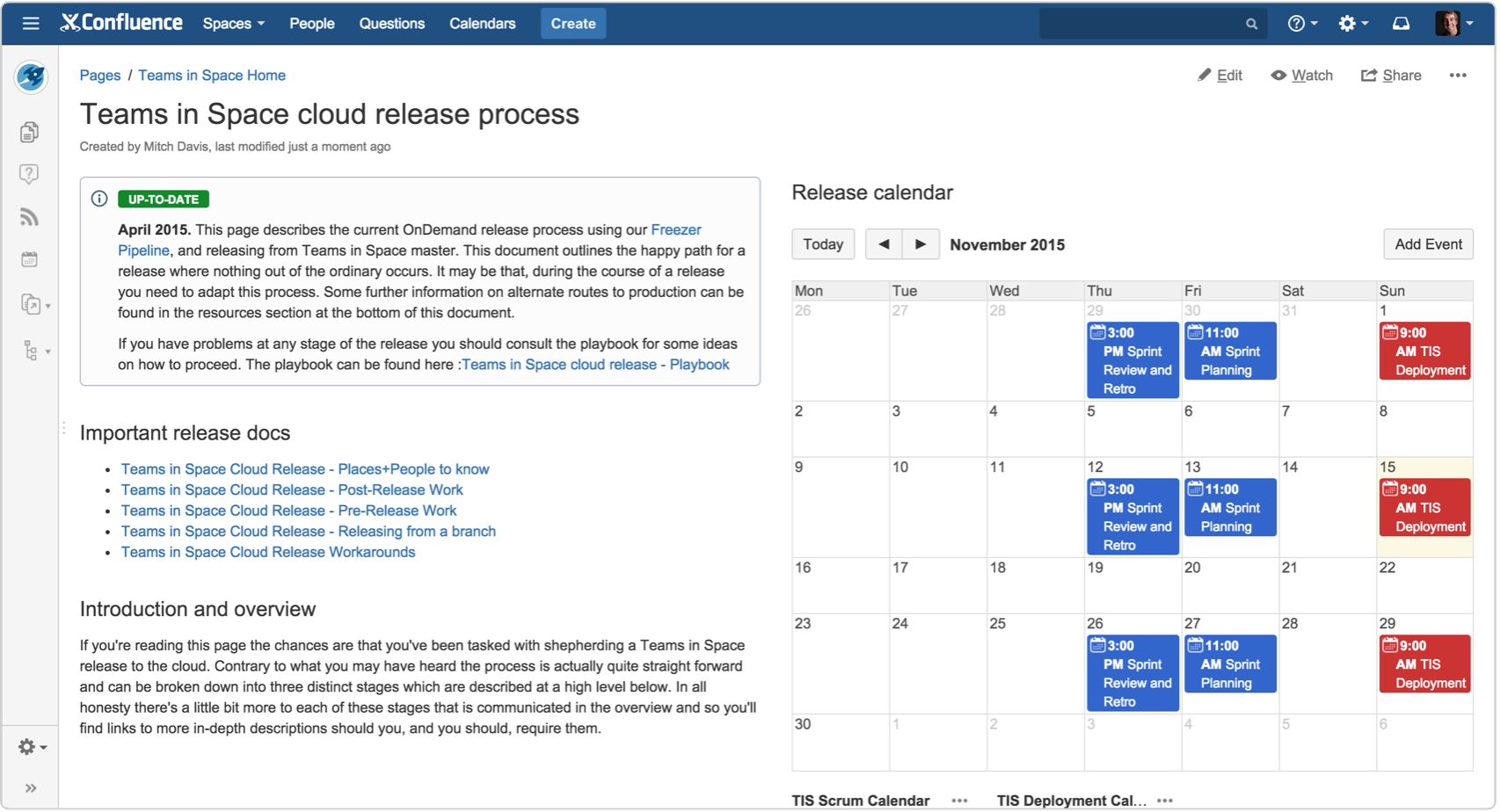The image appears to be a detailed screenshot of a Confluence page against a dark blue background. At the top of the image, the title "Confluence" is prominently displayed. Below the title is a navigation bar with clickable options, including "Spaces," "People," "Questions," "Calendar," and "Create."

Directly beneath the navigation bar, the breadcrumb trail "Pages / Team in Space Home" is shown, indicating the current page hierarchy. The main header in bold black text reads "Team in Space Cloud Release Process." In smaller grey text below, it states "Created by Mitch Davis. Last modified just a moment ago."

Centrally located on the page is a white box with an information icon (a lowercase 'i' inside a circle) to the left, and to the right of this icon is a green rectangle containing the text "Up to Date." Below this section, the text "April 2015" is displayed, followed by a brief explanation: "This page describes the current on-demand release process using our Freezer Pipeline and releasing from Team in Space Master."

Moreover, there is an important note underlined for better readability which clarifies that, "This document outlines the happy path for release when nothing out of the ordinary occurs." Overall, the image provides a clear and structured overview of an on-demand release process within the Confluence platform.